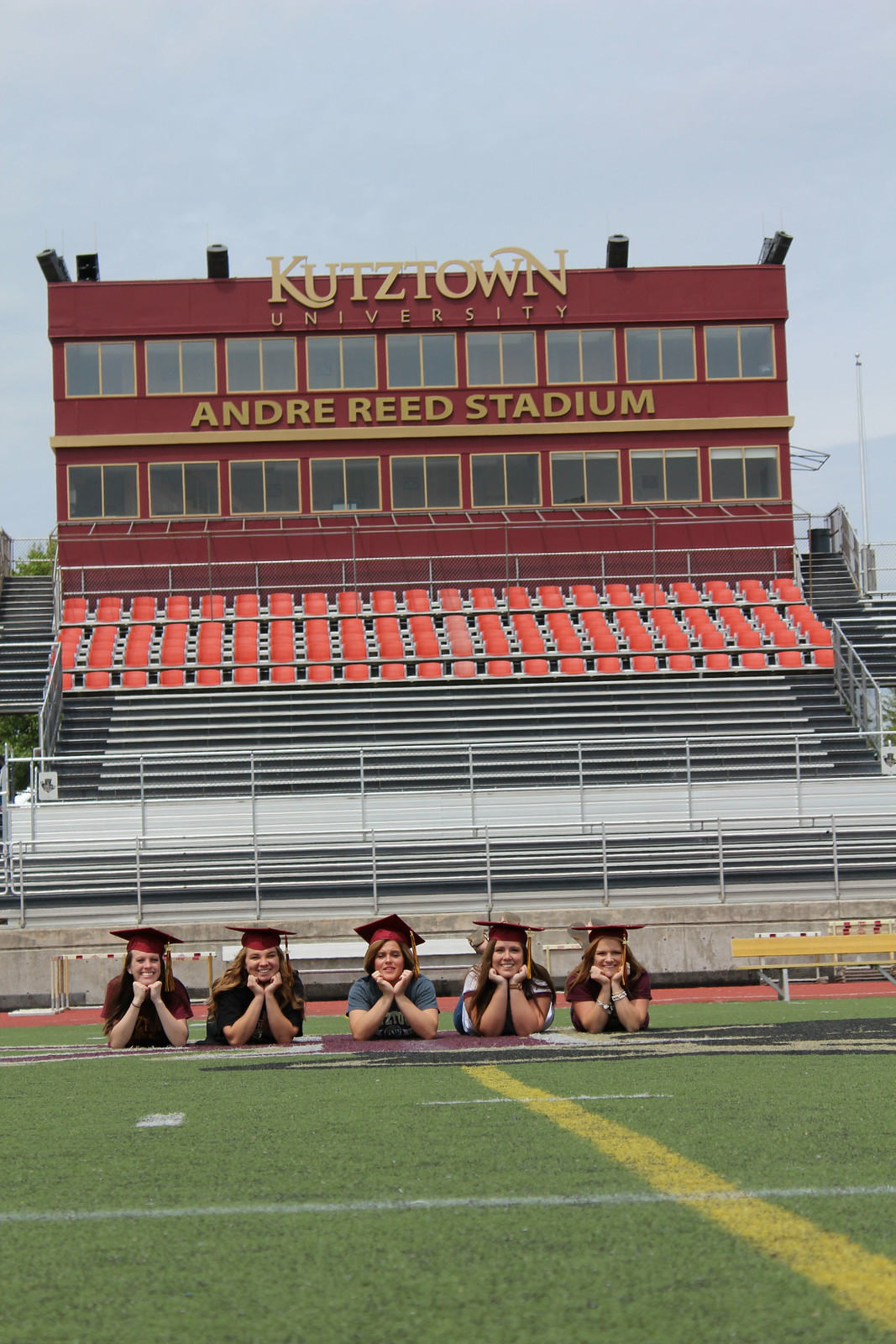The photograph captures five smiling women lying on a football field, dressed in graduation caps that are burgundy and black, with yellow or gold tassels. They are positioned in a row on their chests with their hands under their chins. Behind them, the Kutztown University Andre Reed Stadium dominates the background, featuring a red building with yellow lettering and numerous black windows. The large bleachers in the stadium have orange-colored seats with silver stands. It's a cloudy, overcast day, and a few trees are visible to the left of the stadium. The women are wearing a variety of t-shirts: three in black, one in blue, and one in white. The woman positioned in the center stands out with her blue short-sleeved shirt.